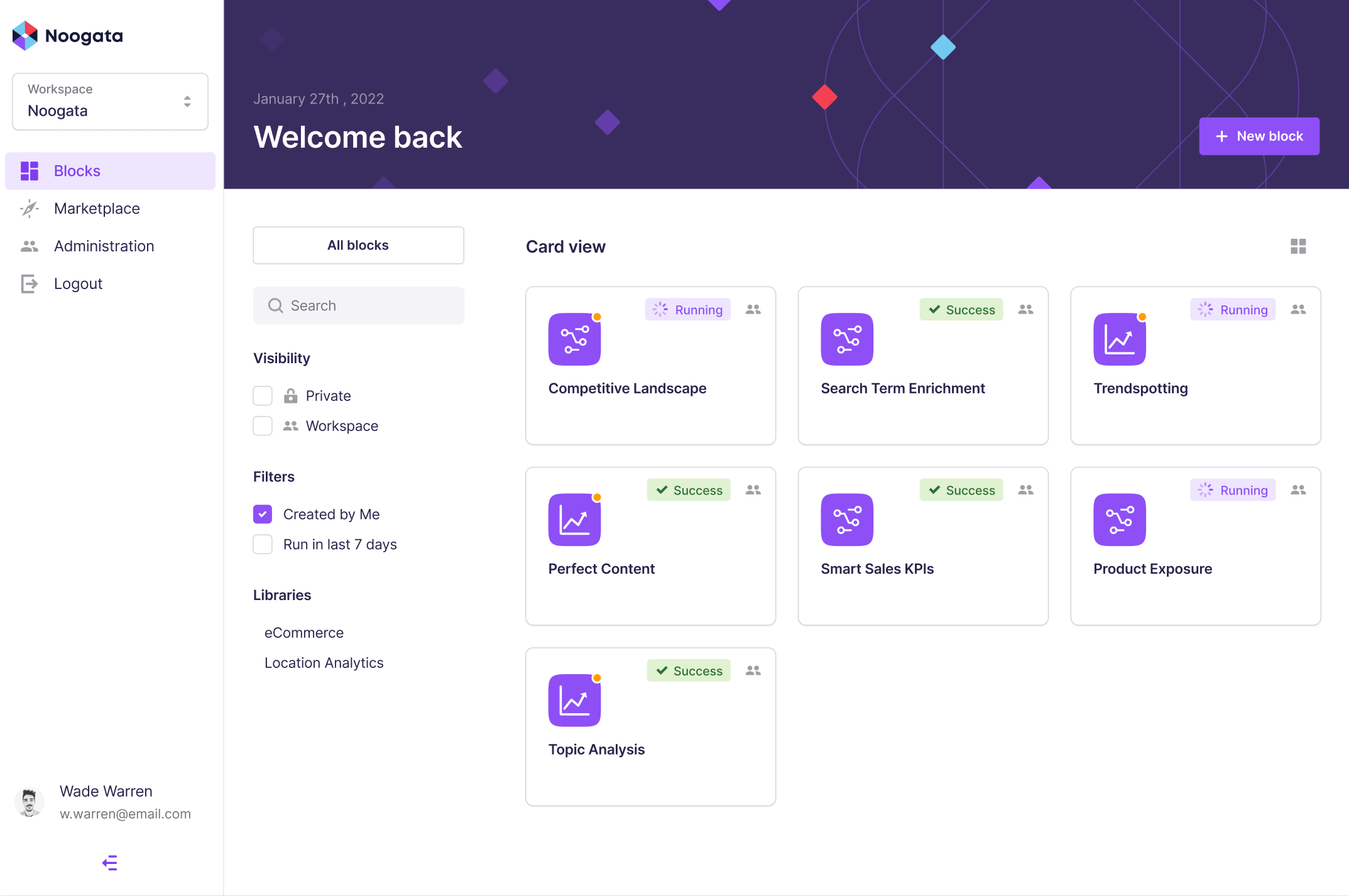The image portrays a detailed and vibrant dashboard interface divided into distinct sections. On the left-hand side, a small horizontally-oriented purple section rises, labeled "Workspace Nogata" in a box with a purple highlight. This highlight emphasizes blocks, also in purple. Directly below, there is another block marked "Marketplace," also associated with Nogata.

In the top part of the image, on the opposite side of a line, a variety of diamond-shaped squares in different shades of purple and red are featured, creating a visually striking pattern. Amongst these, a white text reads "GMWay 27, 2022, welcome back" on the left-hand side. Adjacent to this, a purple rectangle with a white plus sign is labeled "New Block."

Below this, a left-hand column lists options such as "Old Blocks," "Visibility," and "Primary Workspace," with various filters available, marked with checkmarks beside options like "Created by Me," "Libraries," "eCommerce," "Location," and "Analytics." At the bottom of this column, the term "Card View" is prominently displayed.

The main workspace features an organized list of blocks:
1. **Competitive Landscape**
2. **Search Term Enrichment**
3. **Transpotted**
4. **Perfect Contact**
5. **Smart Sales KPIs**
6. **Product Exposure**

Each block is visually separated, culminating in a singular row that contains the "Topic Analysis" box, standing distinctively on its own. The overall interface is designed to enhance user engagement and clarity with a combination of vibrant colors and organized sections.